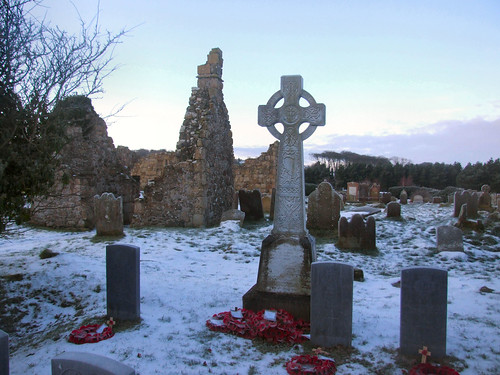The image depicts an old, snow-covered cemetery dominated by weathered headstones. The scene features approximately 25 gravestones scattered across a snowy lawn, indicating a cold winter day. Most notable among the headstones is a tall Celtic cross with a circle around it, suggesting an ancient heritage, possibly Irish.

In the left portion of the image stands a nearly bare tree, a further testament to the wintry conditions, while red commemorative flowers lie at the base of one gravestone. In the backdrop, ruins of a building are visible, comprising mostly fragmented walls and a foundation, lending an eerie, historic atmosphere. The sky above alternates between patches of turquoise blue and thick gray clouds, emphasizing the cold, somber mood. Trees line the distant horizon, completing this evocative and melancholic winter scene.